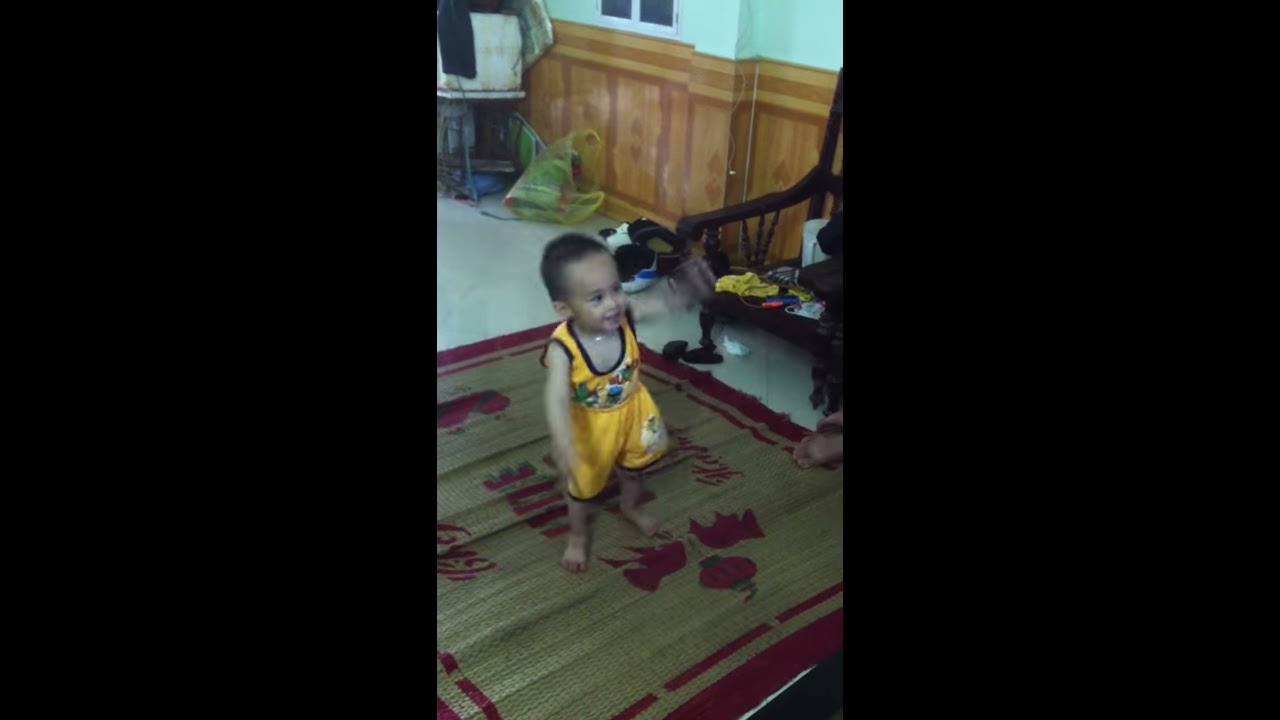In the center panel of the image, a young child, around two or three years old, stands joyfully on a bamboo mat with red trim, which is placed on a light-colored floor. The child, dressed in a matching yellow sleeveless tank top and shorts, exhibits an adorable smile and short, dark hair, while lifting one arm as if in mid-dance. Around their neck is a small necklace. In the background, a wall with wooden paneling on the lower half and white paint above forms the backdrop. To the right, a dark brown wooden chair, cluttered with various objects such as clothes, prevents it from being used for seating. Behind the chair, the bottom half of a person’s foot is visible, indicating someone is sitting and possibly engaging with the child. Further details include a table with items in the upper left corner and a yellow bag on the floor. The scene also features a teddy bear near the child and vents on the upper part of the wall.